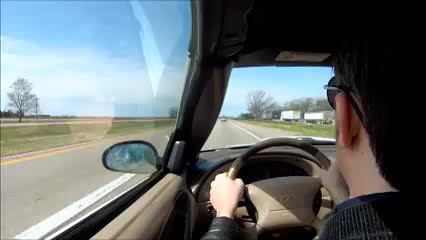The photograph captures the perspective of a driver in a left-hand drive vehicle, wearing sunglasses, navigating a highway on a bright, sunny day under a vivid blue sky. On the right-hand side of the image, another highway can be seen in the distance, populated by what appear to be large white trucks or possibly houses, with trees forming a backdrop. The primary highway is flanked by grass on both sides, and an uninterrupted white line runs along the left edge of the road. Sunlight streams in from the left side, casting a warm glow over the entire scene.